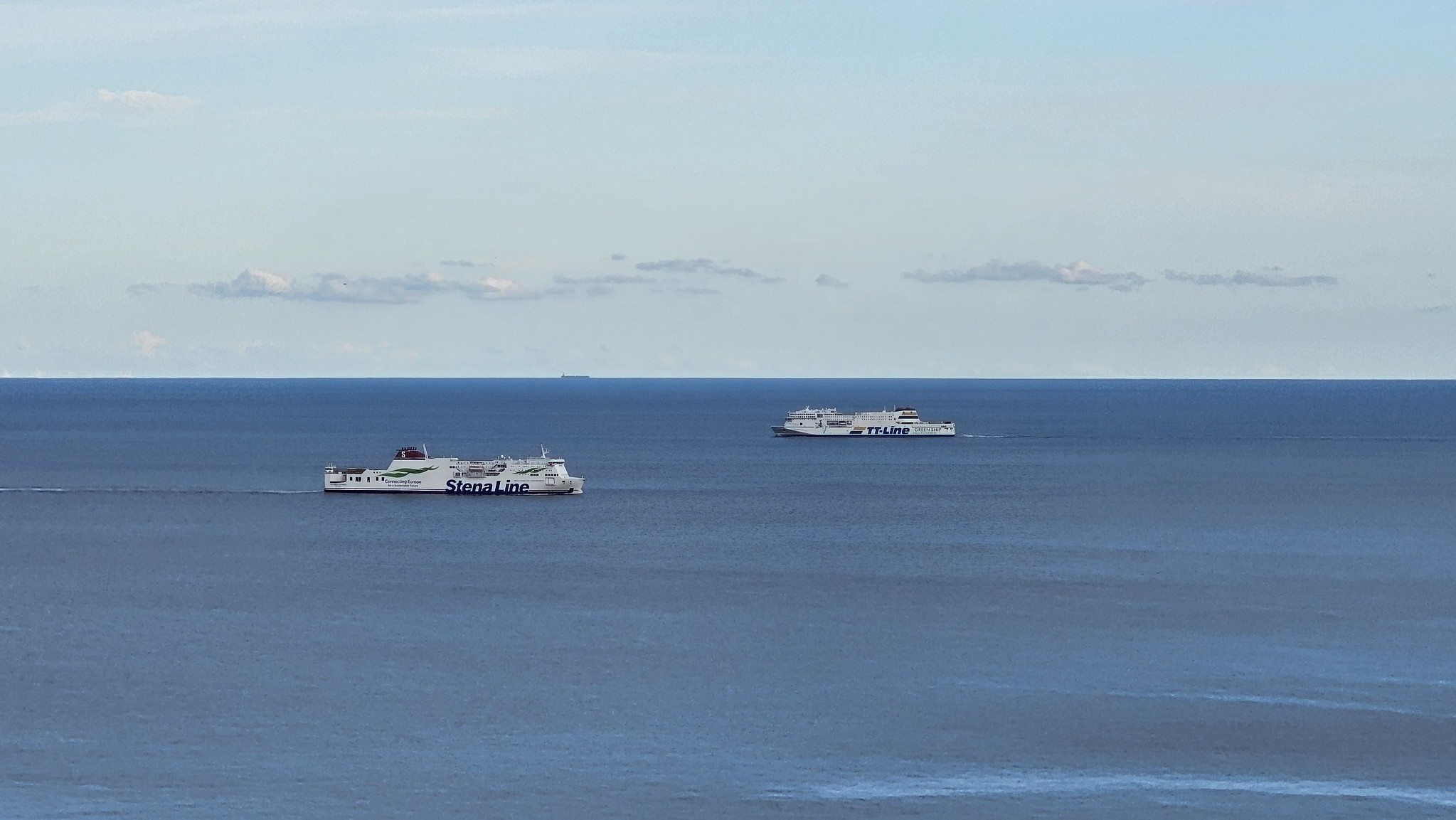This photograph captures a serene seascape featuring two long, white ships sailing on a calm, dark grayish-blue sea. The ship on the left, closer to the viewer, displays the name "Stena Line" in vivid blue letters with a black stack and distinctive black graphics, including a green swishy symbol. This vessel appears to be a multi-deck cruise ship. To the right and further in the distance, the second ship bears the name "TT Line," also in blue letters, accompanied by tan and blue bar graphics. Both ships, devoid of any visible people or cargo, appear small and distant against the expansive backdrop. The horizon stretches across the frame, bordered by a sky that shifts from pale blue to a thin line of dark gray clouds. The overall composition emphasizes the tranquility of the scene, with the ships parallel and slightly displaced, enhancing the sense of depth and distance in the photograph.